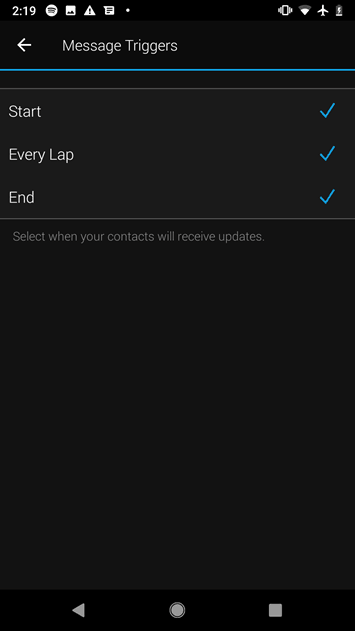The smartphone screen displays a user interface section labeled "Message Triggers" at the top left, highlighted by a horizontal blue line underneath. This section is accentuated by a large white button adjacent to the text. The background of the image is black, creating a strong contrast with the white and gray text displayed throughout.

Below the blue line, a gray line separates the section containing three key words related to message triggers: "Start," "Every Lap," and "End." Each of these words is aligned to the left with a corresponding blue checkmark icon positioned to their right. The interface design features another gray line below these options.

Further down, there is an instructional text in gray which reads, "Select when your contact will receive update." At the very top of the image, the typical smartphone status icons are visible in white, including the current time (2:19), Spotify, gallery, message notification, alert, vibrate, Wi-Fi, airplane mode, battery percent, and battery icon, altogether indicating various active settings and notifications.